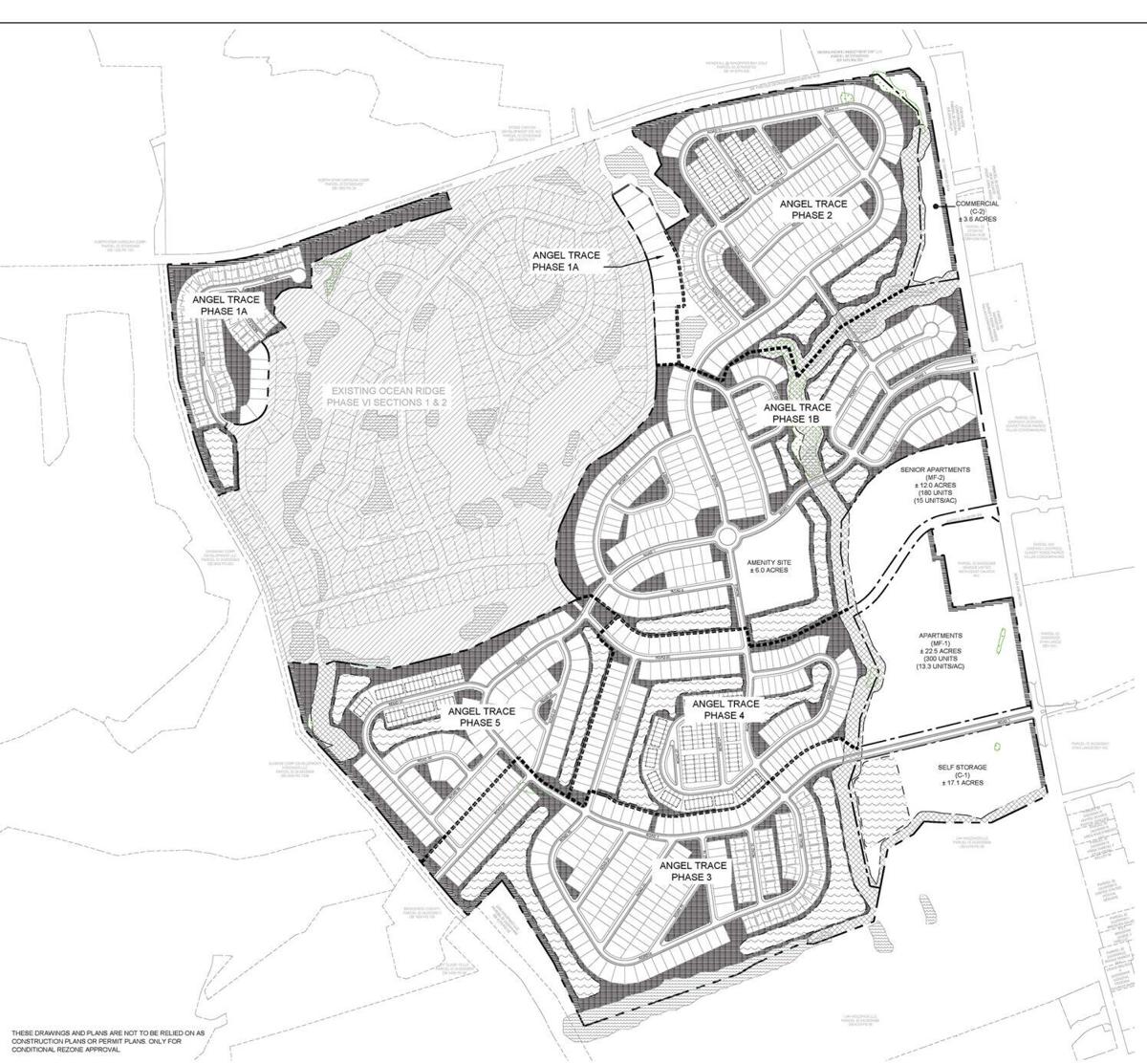This black and white overhead map is a highly detailed blueprint for a planned residential development. The map includes multiple labeled phases of single-family homes, with rows of adjacent homes weaving in and out from each other. Notably, it starts with "Angel Trace Phase 1A" in the top corner, followed by "Angel Trace Phase 2" to the right, continuing sequentially through "Angel Trace Phase 5." Surrounding the clusters of homes are areas designated for additional amenities: a large white geometric area to the right is marked for future apartments, while above it a similar shape is reserved for senior apartments. To the bottom right, a self-storage area is indicated. The plan also includes street views and side streets interspersed between the housing clusters. Sections with existing developments are shaded in gray, contrasting with the white and dark gray areas indicating future projects. Additional, albeit unreadable, text is situated at the bottom left corner of the map, likely providing further details about the development.